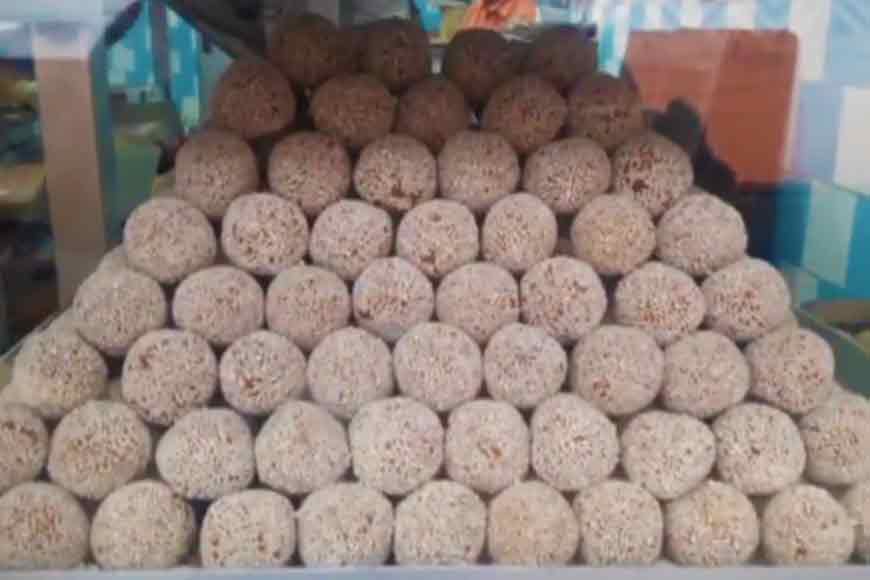An up-close photograph captures the rich texture and inviting appearance of truffles displayed in a bakery's glass case. The truffles, each about the size of a ping-pong ball but appearing much larger due to the close perspective, are meticulously arranged in rows on a tray, resembling the size of baseballs in the image. They boast a light Dutch cocoa color, having been generously dusted with cocoa powder, revealing glimpses of the decadent, darker chocolate beneath. 

In the background, the bakery's decor comes into view, featuring a checkerboard pattern on the wall with alternating squares of light and deep blue hues. To the left, another glass case is partially visible, characterized by a taupe leg and bar, and topped with white. Inside this case, shelves are lined with items in various colors including white, yellow, and brown, adding to the vibrant confectionery display. The back wall is adorned with a painted red gift-style bag and a hanging poster, completing the cozy, inviting atmosphere of the bakery.